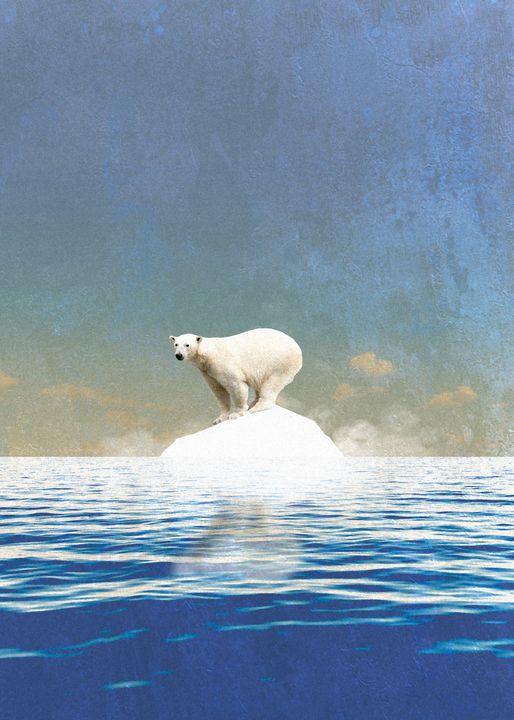This is a detailed digital rendering of a solitary polar bear stranded on a small, irregularly shaped iceberg in the middle of a vast ocean. The bear, off-white in color, clings to the iceberg with its head facing left and its hindquarters to the right. Reflections of both the polar bear and the iceberg ripple across the blue ocean waters, which are highlighted with white accents and dappled with sunlight glint. The sky provides a striking backdrop, transitioning from a light blue-gray at the top to a yellowish-tan closer to the horizon, interspersed with hints of white and light brown clouds. The image, vertically aligned and possibly resembling a painting, captures the poignant isolation of the bear against the ethereal expanse of sky and sea.